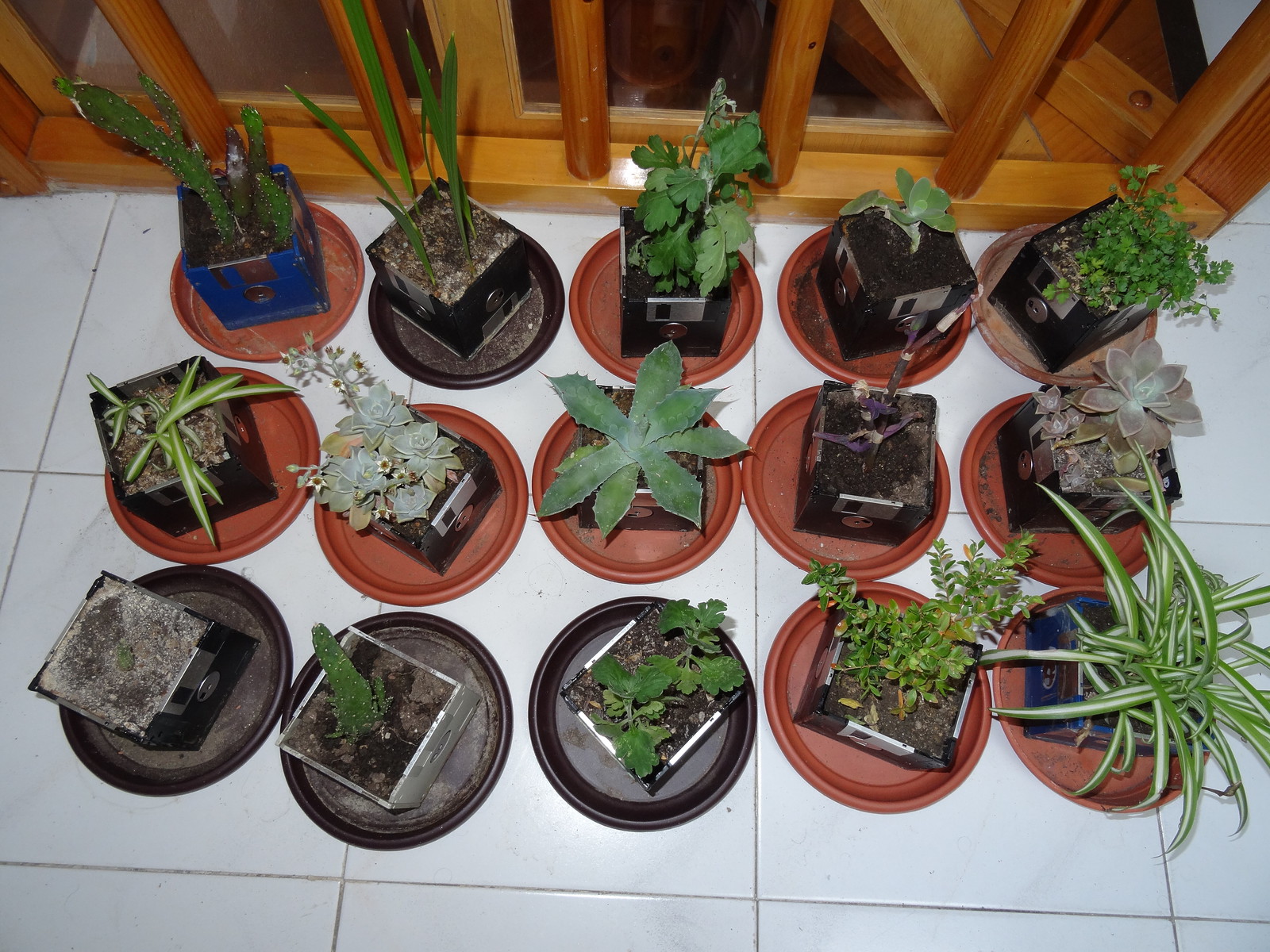This image captures 15 potted plants meticulously arranged on the large, white, square-tiled floor of what appears to be someone's house. The plants are organized in five vertical rows of three, each plant housed in a short, square pot. These pots rest on round bases, primarily terracotta in color with some exceptions; specifically, the bottom left corner has three plants set on black trays. The diversity of the plants is striking, with no two plants appearing the same. On the bottom right, a particularly wild plant features long, unruly strings of leaves splaying out in various directions. The middle row contains plants with more orderly, straightened leaves, presenting a conventional appearance. Meanwhile, the bottom left features a struggling small sprout, seemingly on the verge of failing to grow. Among the collection, there are various succulents, a cactus in the upper left, a clover-like plant in the upper right, and even a uniquely pale purple plant. Overall, the greenery thrives in an array of clay dishes, adding a touch of nature to the orderly indoor setting.